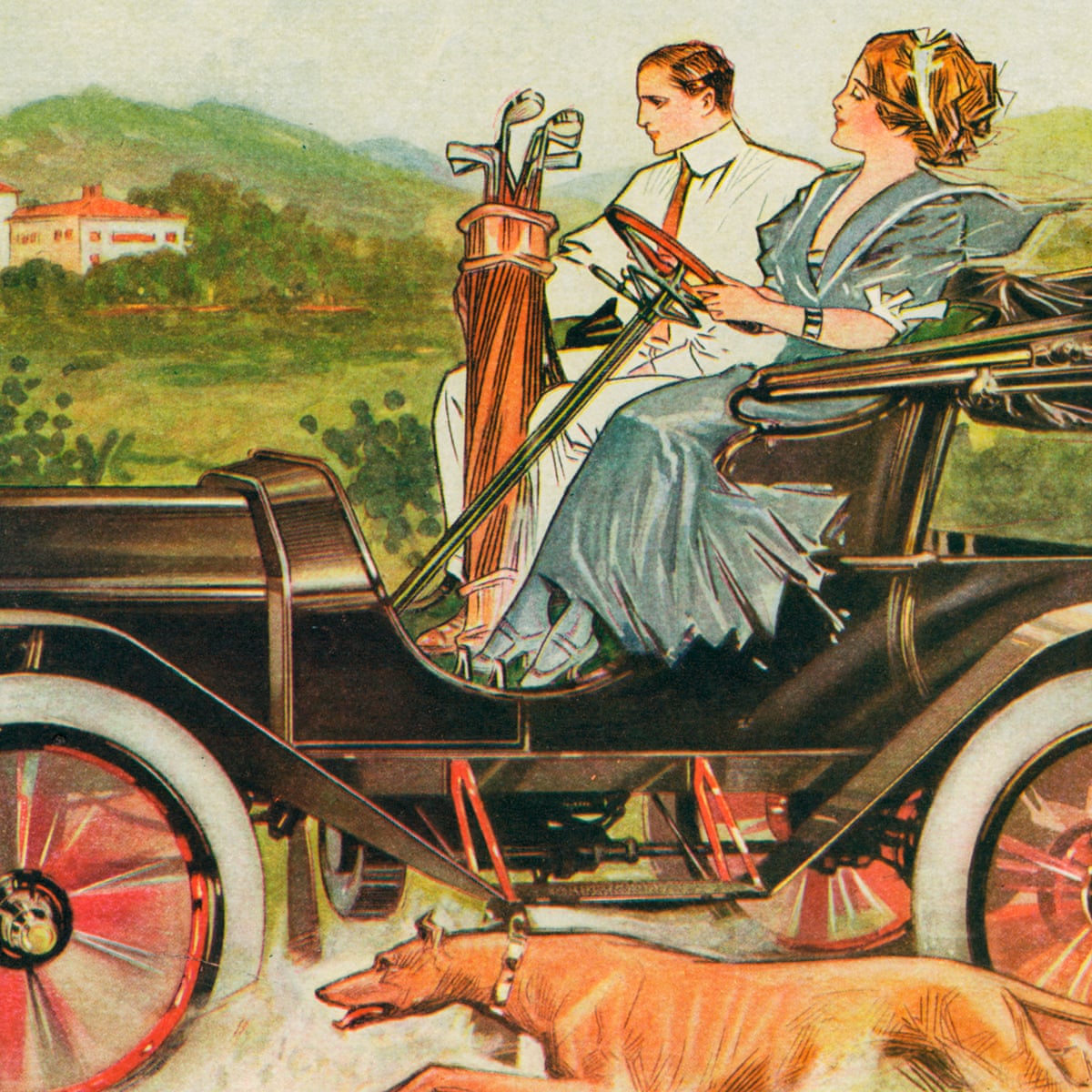This detailed illustration, reminiscent of an old-timey book or magazine, features a scenic backdrop of green mountains, trees, and a white house with a red roof nestled in the background. At the forefront, a man and woman ride in a vintage, black carriage-like vehicle with distinctive white wheels and red rims. The vehicle is open-air, showcasing the simplicity of early automobiles, with a tall steering wheel extending from the floor to the woman’s hands. The woman, adorned in a blue dress with a ribbon in her blonde hair, is driving. Beside her, the man, donned in a white dress shirt, white pants, and a white tie, holds onto his golf clubs encased in an orange bag. A brown dog runs alongside the car, adding a touch of liveliness to the serene, illustrated scene.